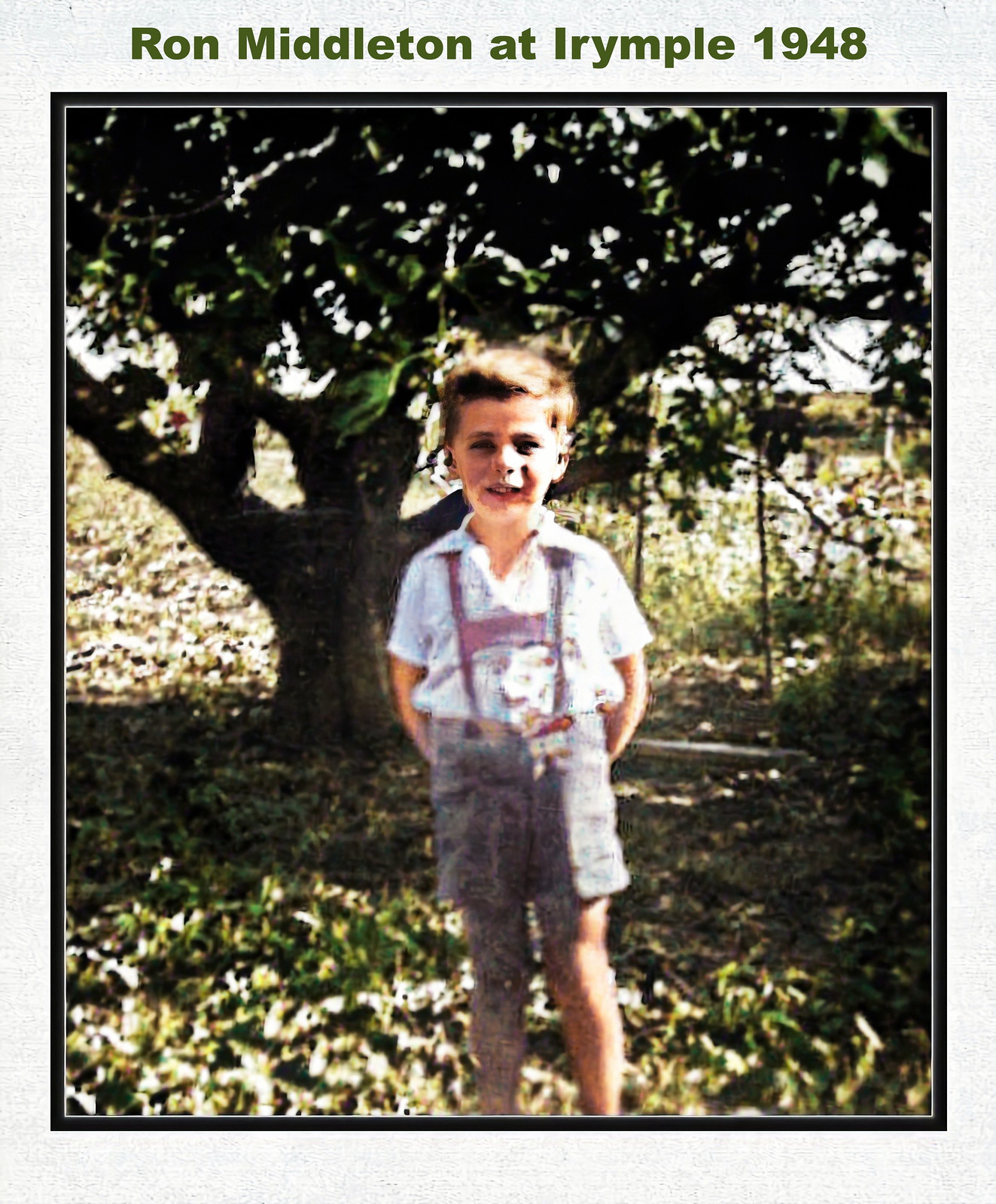This is a colorized photograph from 1948, depicting a young boy named Ron Middleton. The photo itself is framed by a gray border, with a caption at the top in green or dark green text reading "Ron Middleton at Irymple 1948." The boy appears to be around five or six years old and is posed standing in front of a large tree with green leaves, with green grass and some fallen leaves underneath him. He has brown hair and wears a button-up white shirt paired with gray lederhosen. His lederhosen have straps that go over his shoulders and connect at the back. The boy stands with his arms partially behind his back, giving a slight smile. The image, although blurry due to its age, captures a serene moment in a shaded outdoor space.